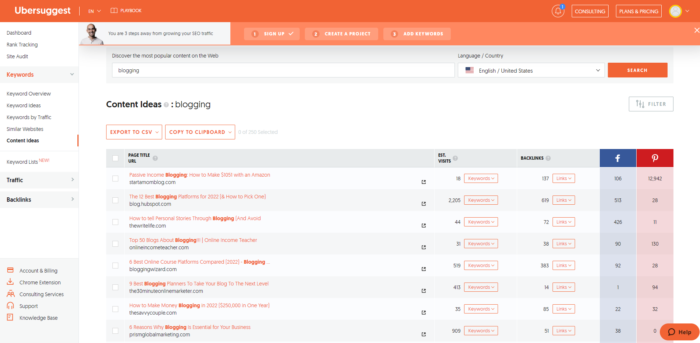**Descriptive Caption:**

A screenshot of the UberSuggest website interface is depicted. The top section features a prominent orange banner with the words "UberSuggest" displayed in white font. Adjacent to this, text that reads "Plans and Pricing" appears within the same vibrant orange background. Below this banner, an image of a person is visible, accompanied by a partially legible message stating, "You are three [words unclear] away from getting your $40 [words unclear]." Beside this image are buttons labeled "Sign Up," "Create a Project," and another unspecified button.

On the left side of the interface, a vertical menu is presented against a white background. The menu items, written primarily in black with select text in orange, include "Dashboard," "Tracking," "Site Audit," and "Keywords" (the latter being highlighted in orange). Further menu items are listed in black bold text: "Keyword Overview," "Keyword Ideas," "Traffic," and "Backlinks." Subcategories under these headings read "Accounts & Settings," "Chrome Extensions," "Support," and "Knowledge."

The central portion of the interface showcases "Content Ideas—Blogging." This section appears to list various blogging articles, although the titles are too blurred to discern. Engagement indicators such as "Wow" (possibly associated with social media platforms like Facebook and Pinterest) and numerical data related to "backlinks" are also present, though specifics are obscured.